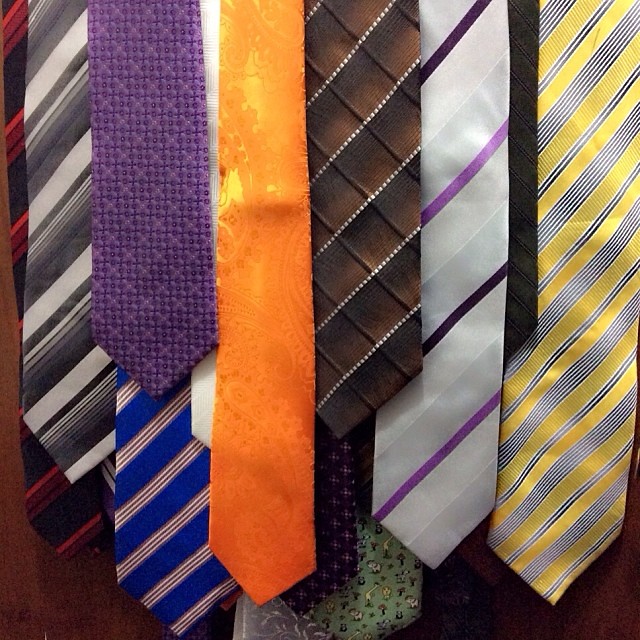This image features a close-up of various men's neckties, neatly hanging with their points facing down. In the foreground, a prominent yellow silk tie with blue and white grouped stripes catches the eye with its glossy sheen. To the right of this tie, a small edge of a plain dark tie, possibly brown or black, is visible. Draped over this is a tie with purple, gray, and darker purple stripes. Moving left, a brown tie with shaded squares and white dotted lines stands out. Next to this, a slightly frayed plain orange tie is positioned, followed by a purple tie adorned with light purple dots.

Adjacent to these, another tie features gray and white stripes. Background ties, less visible but present, include various red, black, and blue striped options along with some green and brown ties. There's mention of a white tie with black stripes and another black tie with red stripes in the mix, adding to the diverse collection of colors and patterns showcased. The neckties vary in width, with thinner ties in front and wider ones towards the back, forming a layered, textured display of classic men's accessories.